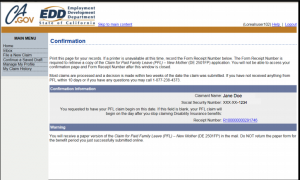The screenshot depicts an official California government website, identifiable by the distinct header at the top. The background is primarily white. In the upper-left corner, the logo "CA.gov" features the letters "CA" styled in a blue, handwritten font, while ".gov" appears in gold. Next to this, the acronym "EDD" is prominently displayed in dark blue capital letters. Below "EDD," the full title "Employment Development Department" is written, each word on a separate line in blue font. Underneath these elements is a gold line, matching the color of ".gov" in the logo.

Along the left side of the screenshot is a sidebar. The top third of the sidebar is a medium grayish-blue, and the remainder transitions to a lighter blue. The text within the sidebar, although largely illegible due to size, includes a heading labeled "Main Menu."

Central to the image, towards the top left, the word "Confirmation" appears in a blue font. Beneath this are several unreadable paragraphs of text. A blue line separates these paragraphs from the next section, which features a background in a medium blue-gray color. This section also contains text that is too small to decipher. Following another blue line, the remainder of the website's content is displayed on a white background containing about one and a half lines of nearly unreadable print.